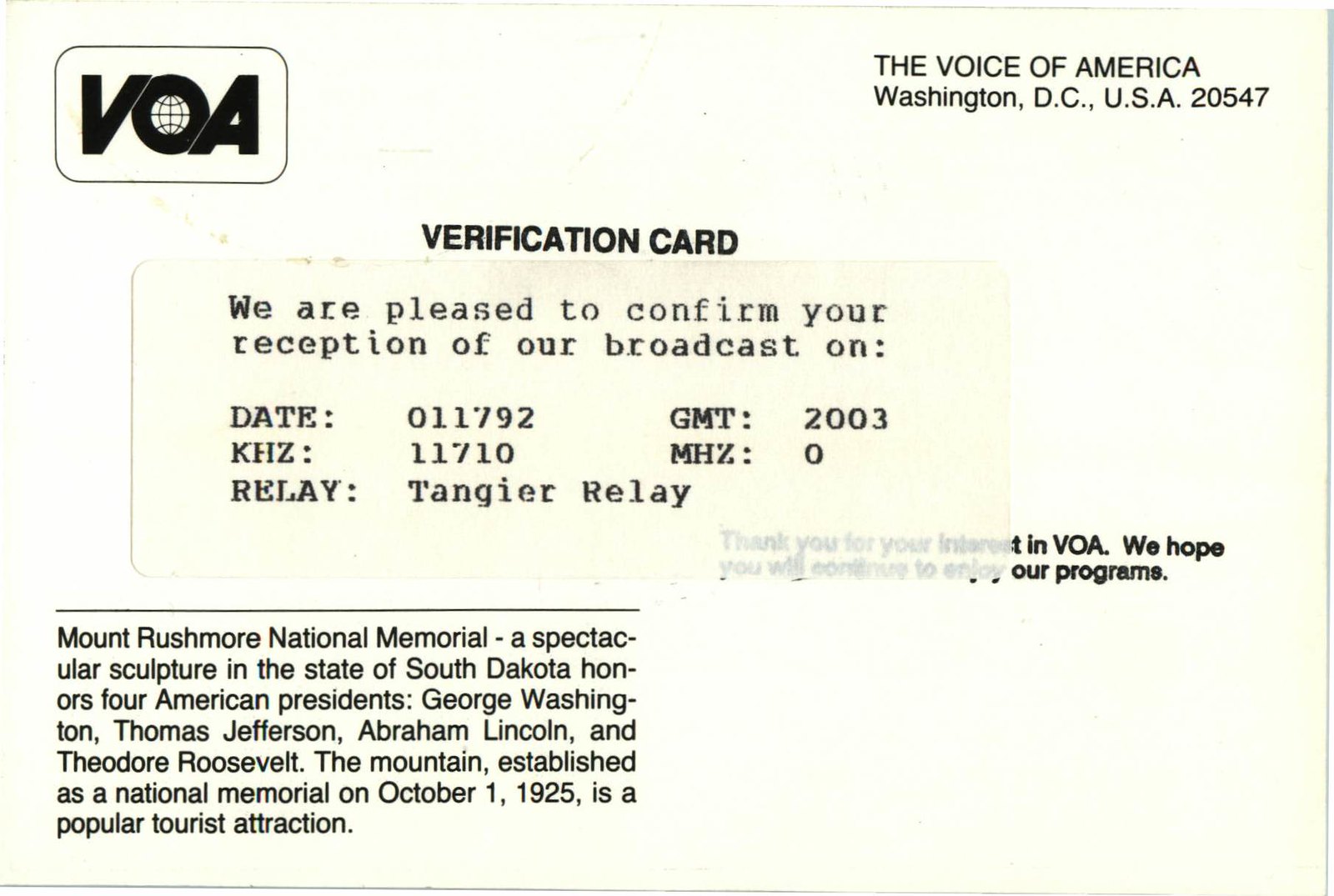The image is a horizontal, rectangular verification card with a yellowed off-white color. In the top left corner, there is a VOA logo, featuring a globe with latitude and longitude lines inside the 'O'. The top right corner contains the text: "The Voice of America, Washington, D.C., U.S.A., 20547". Centered in larger type, the card reads "Verification Card", with a sticker below, stating: "We are pleased to confirm your reception of our broadcast on," followed by specific date and frequency details. The lower left side features a descriptive paragraph that begins with "Mount Rushmore National Memorial," describing the memorial as a spectacular sculpture in South Dakota that honors Presidents George Washington, Thomas Jefferson, Abraham Lincoln, and Theodore Roosevelt. It notes that Mount Rushmore was established as a National Memorial on October 1, 1925, and is a popular tourist attraction. The verification card is white with black writing and has notable text placements.